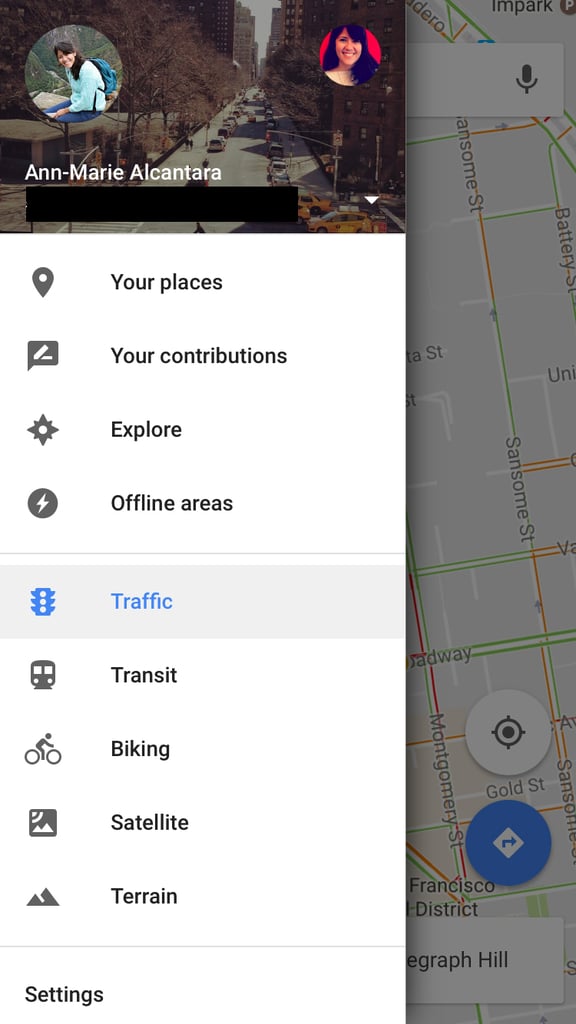The image is a vertically oriented rectangle. In the top-left corner, there is a circular frame containing the side profile of a woman with long hair, facing left. In the upper right corner, there is a smaller circle featuring the same woman, this time looking straight ahead. The background of the upper horizontal rectangular area depicts a city street viewed from above, at a distance.

Below this scene, the name "Anne-Marie Alcantara" is displayed in bold white font. Beneath it, a black horizontal rectangle appears to obscure some information. Below this black rectangle, on the left side, there are some logos, while on the right side, black bold text on a white background reads: "Your places, Your contributions, Explore, Offline areas."

Following this, in a light gray rectangular area, blue text and icon indicate "Traffic." Further down, black text lists: "Transit, Biking, Satellite, and Terrain." A light gray horizontal line separates these sections. At the very bottom left corner, the word "Settings" is displayed. The lower section of the image partially reveals a map, but its details are not clearly visible.